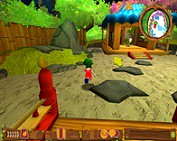This image appears to be a small, pixelated screenshot from an older 3D video game, reminiscent of Nintendo 64 graphics with a very small dimension, roughly 1.5 inches by 1.5 inches. The scene seems to be set in a Japanese-inspired environment, featuring an open-air structure resembling a pagoda or Asian-style temple in the background. This structure showcases a distinctive wooden frame and a curved, tile roof that curls up at the edges. 

In the foreground, you are viewing the scene from what appears to be a wooden porch or railing. Below this porch, there seems to be a small panel that could represent the player's inventory and hotkeys. Prominently, there is a character in red attire with green hair, possibly a red dress or cape, moving towards the temple-like structure in the distance. Accompanying this character is another figure, perhaps a child wearing a red t-shirt, blue cap, and blue shorts.

The scene is framed with various environmental details, including a fence to the left, hedges and trees sprinkled around, and a walkway made of large, dark gray stepping stones leading towards the temple. Additionally, there's a mini-map located in the top right corner of the screen, aiding in navigation.